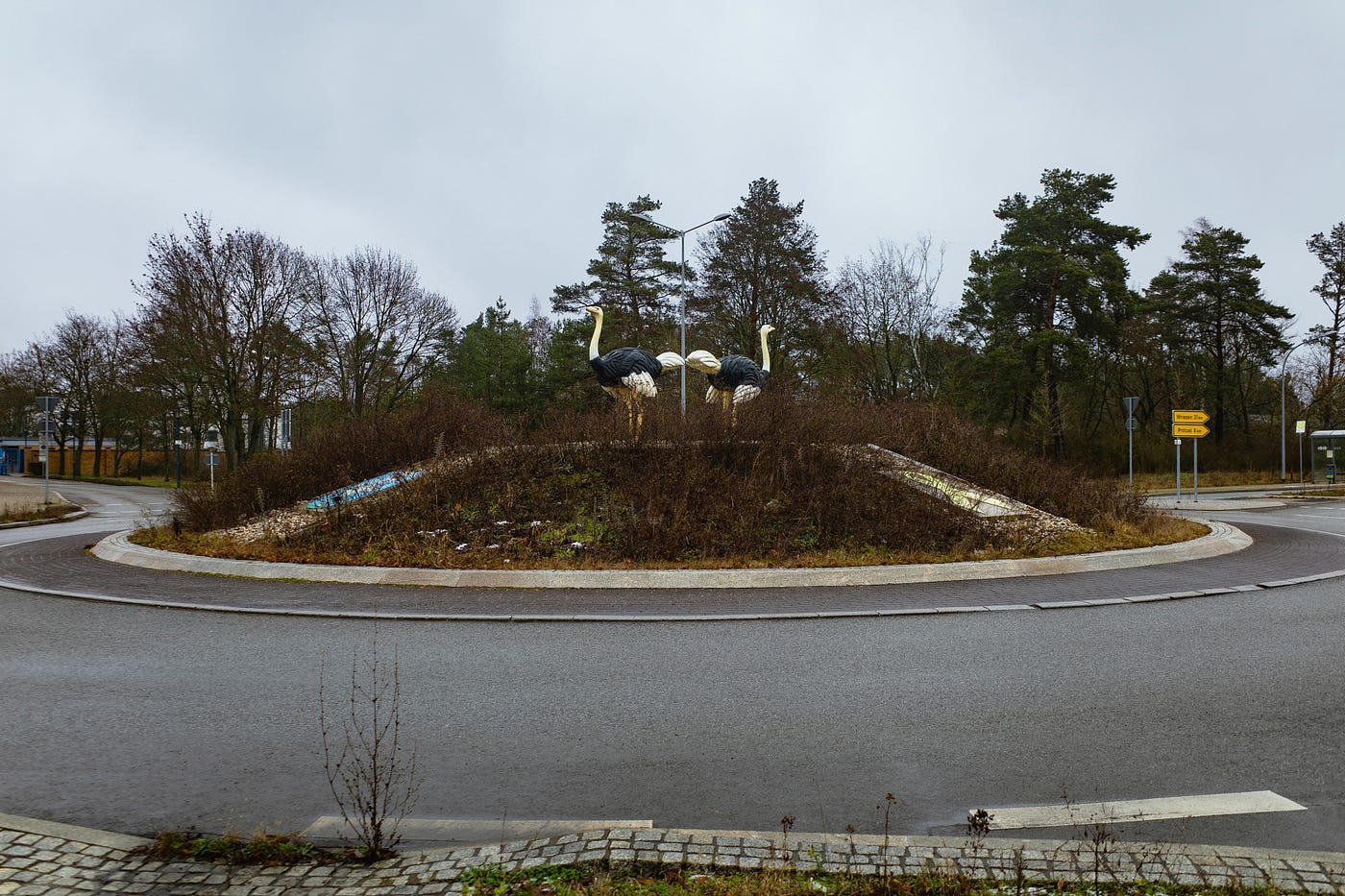The photograph depicts a roundabout, presumably in a European city, with a distinctly landscaped center. The roundabout is characterized by a raised, circular mound bordered by a curb and embellished with several dark brown, twiggy shrubs. Ascending from the street level, which is a dark gray, are walkways and ramps leading to the top of the mound. Prominently situated at the apex are two large, fiberglass ostrich statues. These statues stand back to back, each ostrich poised with heads held high, gazing outward. The ostriches are distinguished by their golden necks, black bodies, white wing and tail feathers, and yellow legs and beaks. Surrounding the roundabout is a verdant landscape featuring a cluster of trees and, visible in the background to the left, structures that give the impression of a suburban setting. Yellow signage points in one direction, enhancing the organized, navigable appearance of this urban roadway feature.